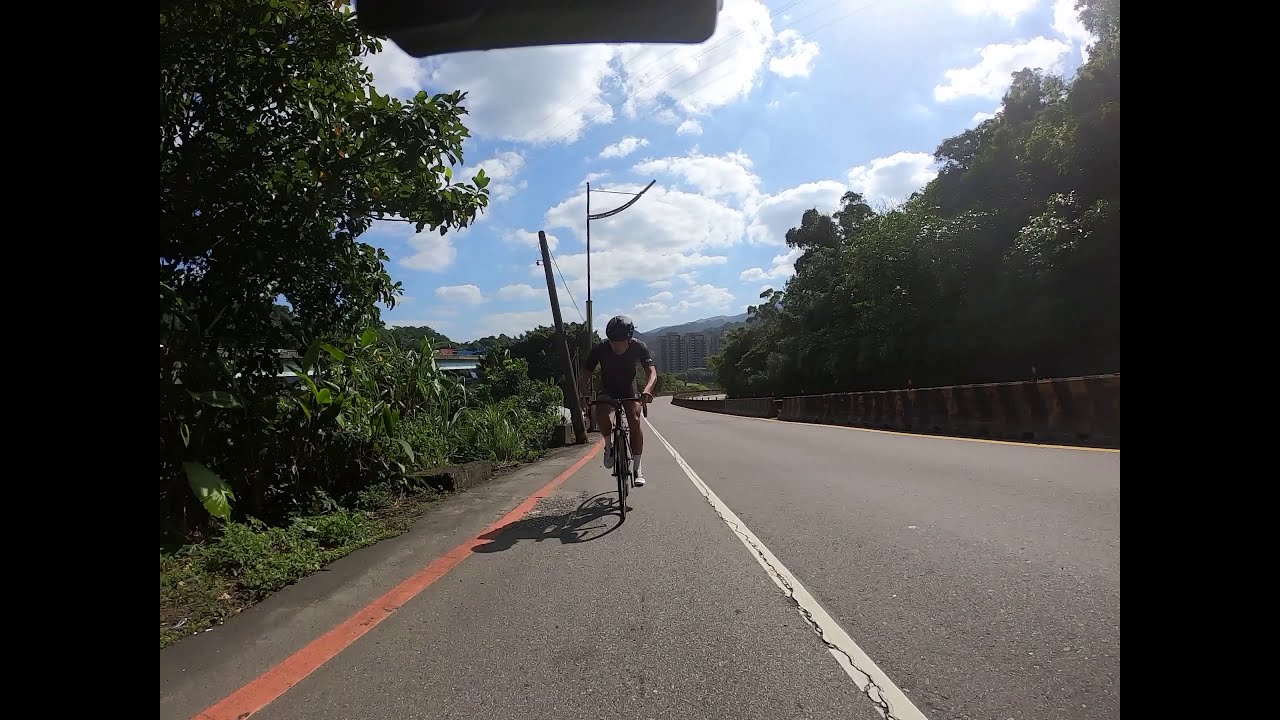The image captures a lone bicyclist riding towards the camera on a quiet road, centered in the frame. The rider, wearing a black helmet, black shirt, shorts, and white shoes, is positioned within a bike lane marked by a solid white line on the right and a dark orange line on the left. Flanking the road on both sides are lush green trees, bushes, and shrubs, contributing to a verdant, natural setting. Behind the bicyclist to the left, a wooden electricity pole with attached wires is visible, and beyond it, a metal pole supports additional cables. Rooftops peek through the trees on the left side, adding an element of tucked-away dwellings. The road curves to the right in the distance, climbing a steep hill with a scenic backdrop of rising mountains. A guardrail or railing runs along the far right of the road, possibly accompanied by a bridge. In the very background, taller buildings are faintly visible against a bright blue sky adorned with fluffy, rounded white clouds. The composition is framed with dark sections on either side of the photo, emphasizing the central bicyclist and the picturesque, serene surroundings.